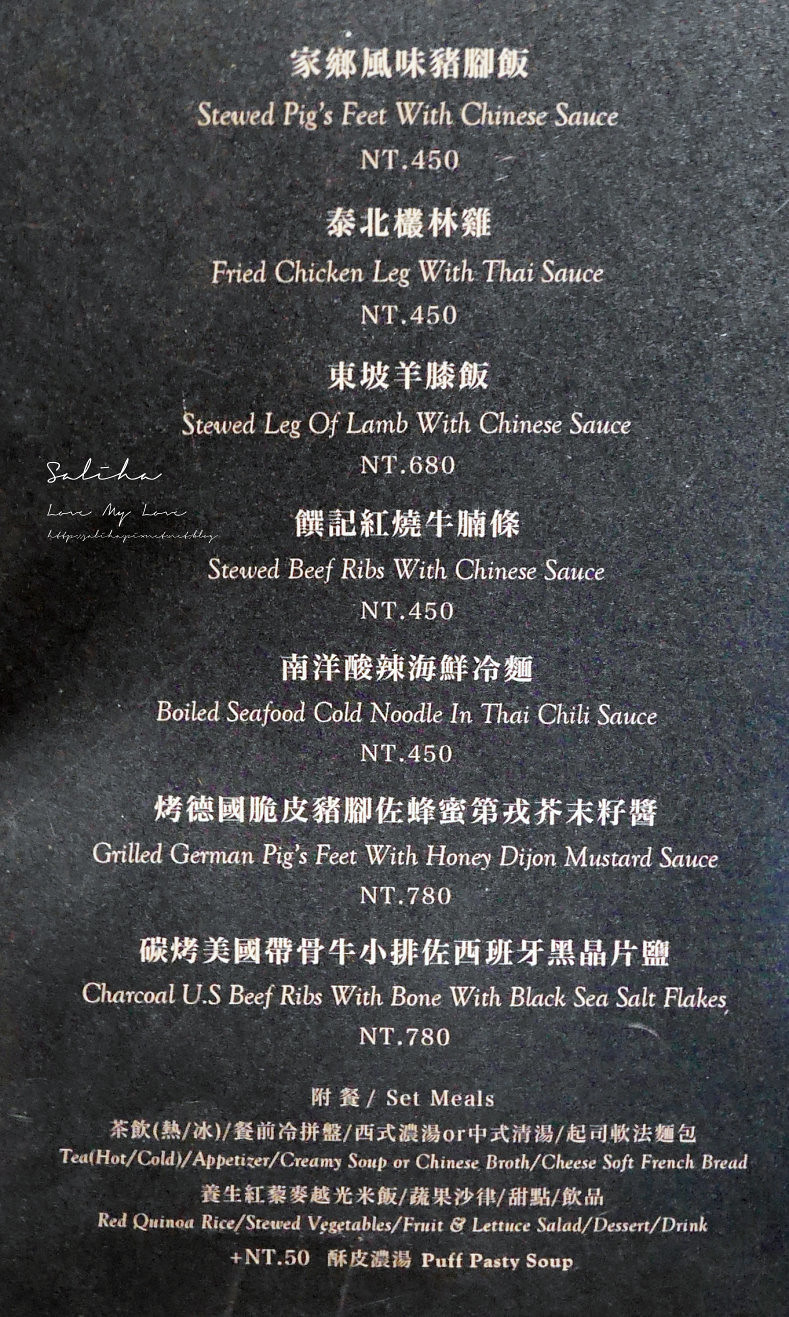In the image, a restaurant menu is prominently displayed against a textured black background that resembles a countertop, speckled with bits of gray and white. The menu is bilingual, featuring an Asian script—possibly Chinese or Japanese—above English translations. The English section lists mouth-watering dishes in descending order: stewed pig's feet with Chinese sauce, fried chicken leg with Thai sauce, stewed leg of lamb with Chinese sauce, stewed beef ribs with Chinese sauce, boiled seafood cold noodle in Thai chili sauce, grilled German pig's feet with honey Dijon mustard sauce, and charcoal U.S. beef ribs with bone accompanied by black sea salt flakes. At the bottom, there's a note explaining that some meal options include tea, an appetizer, soup, bread, stewed vegetables, salad, dessert, and a drink, indicating a comprehensive dining experience.